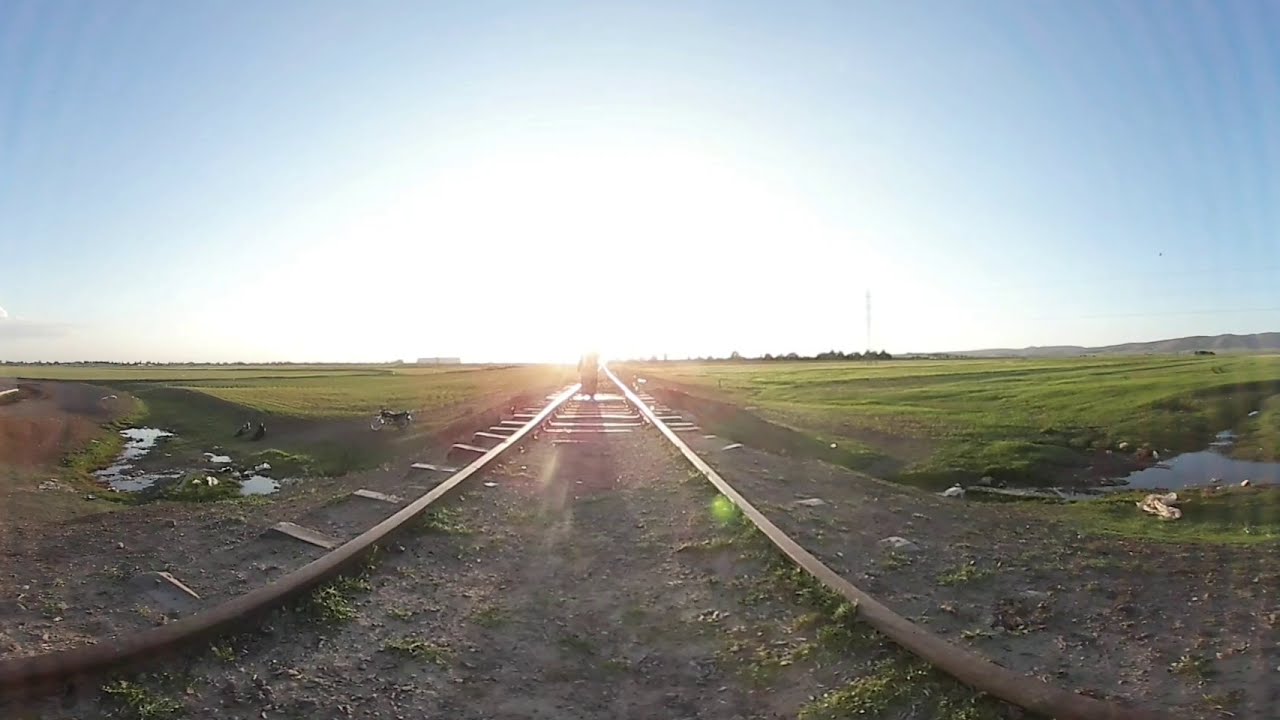The image captures a sunlit, serene countryside scene dominated by an abandoned railroad track veiled in grass and dirt, indicating it hasn't been used in a long time. Centered on the tracks is a person, mostly obscured by the intense brightness of the midday sun that creates a white halo effect, washing out part of their body. To the right of the tracks, there's a small pool of water, while on the left, a few gentle hills can be seen. Two people are sitting on these hills next to a motorcycle. The expansive fields stretch out on both sides, with farmland extending as far as the eye can see, punctuated in the far distance by a few trees and a building. The wide, clear blue sky devoid of clouds blankets the scene, emphasizing the peacefulness of this rural landscape. In the background, a large cell phone or radio tower rises, and faintly behind it, more hills are visible. The scene is bathed in sunlight, enhancing the vibrant green of the fields and contributing to the tranquil, idyllic atmosphere.